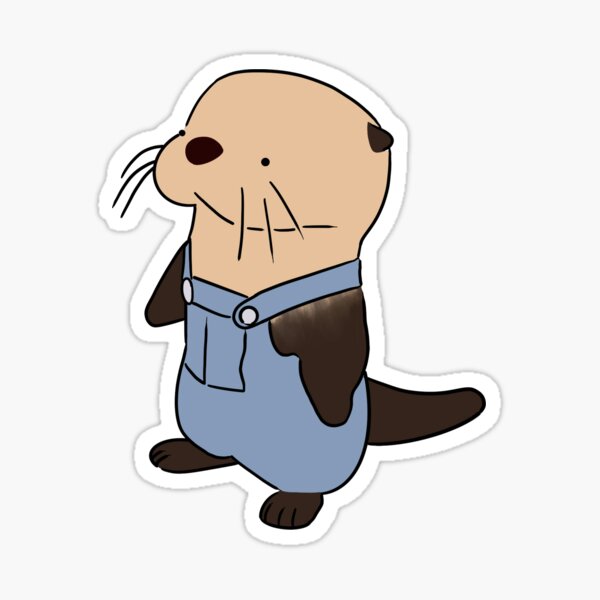This image captures a minimalist cartoon sticker of a young sea otter with a white border, placed on a flat white surface. The otter, resembling a little kid, is looking to the left with a light tan face, small beady black eyes, and dark brown ears and nose. It has three whiskers on each cheek and a slightly grim expression. The otter is dressed in blue overalls with white buttons on the shoulder straps and a small pocket on the front. Its arms, resembling paddles, feet, and long tail are dark brown, sticking out from the overalls. The simple, detailed nature of the cartoon, coupled with the light, neutral background, gives it a distinctive minimalist and somewhat Japanese style.